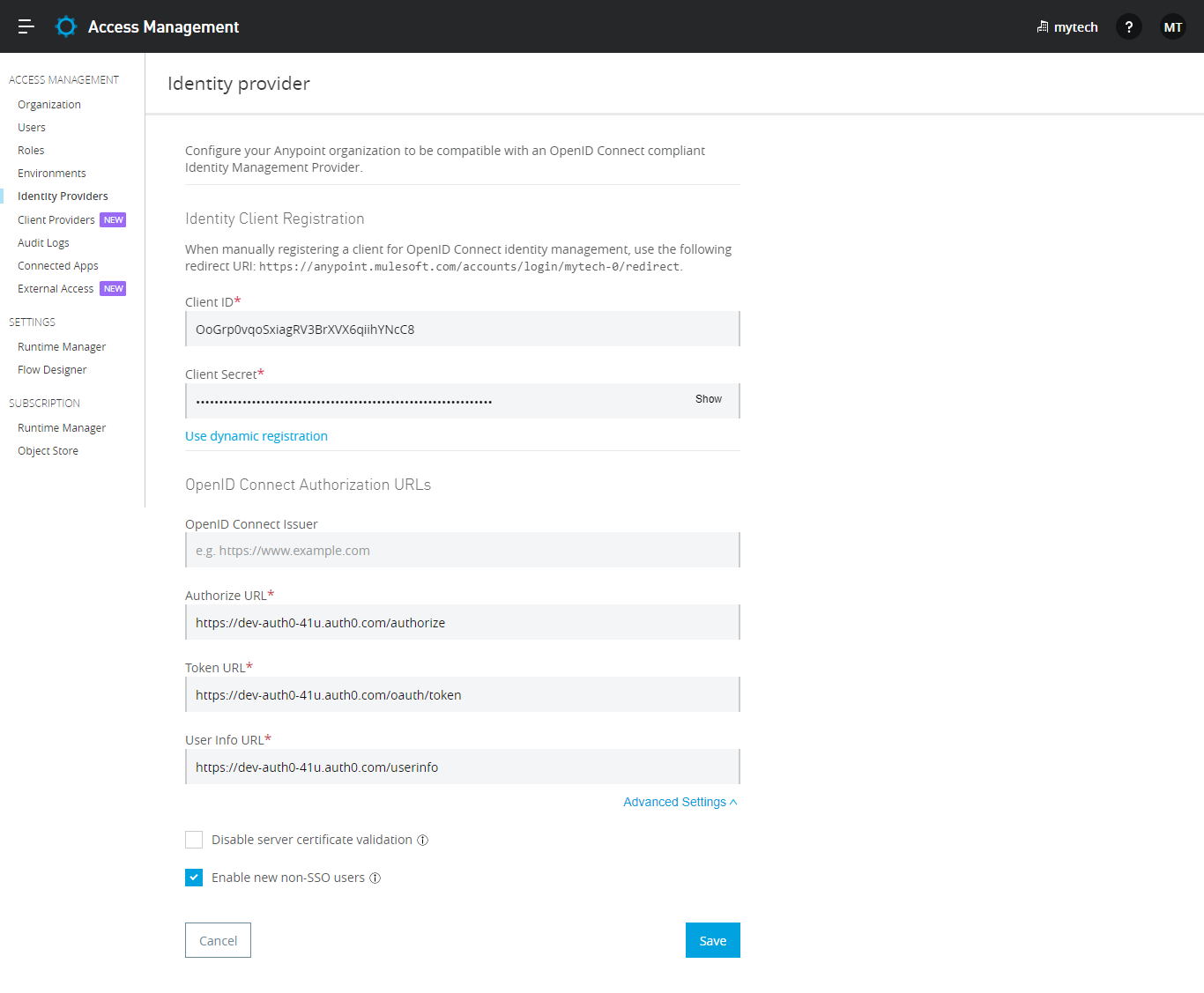A screenshot from an individual's device captures the Access Management page, displaying a comprehensive navigation panel on the left. The panel lists various sections including Organization, Users, Roles, Environments, Identity Providers, Client Providers, Audit Logs, Connected Apps, External Access, Settings, Runtime Manager, Flow Designer, Subscription, and Object Store. Within this list, the 'External Access' and 'Client Providers' sections are highlighted by new, purple labels indicating recent additions or updates. The focus of the screenshot is on the 'Identity Providers' section, which has been selected, revealing a detailed configuration form in the main viewing area. This form allows users to configure their Anypoint organization to be compatible with an OpenID Connect-compliant identity management provider. The form includes fields for the 'Client ID', which has been filled in, and the 'Client Secret', the latter of which is obscured by black dots for security purposes.